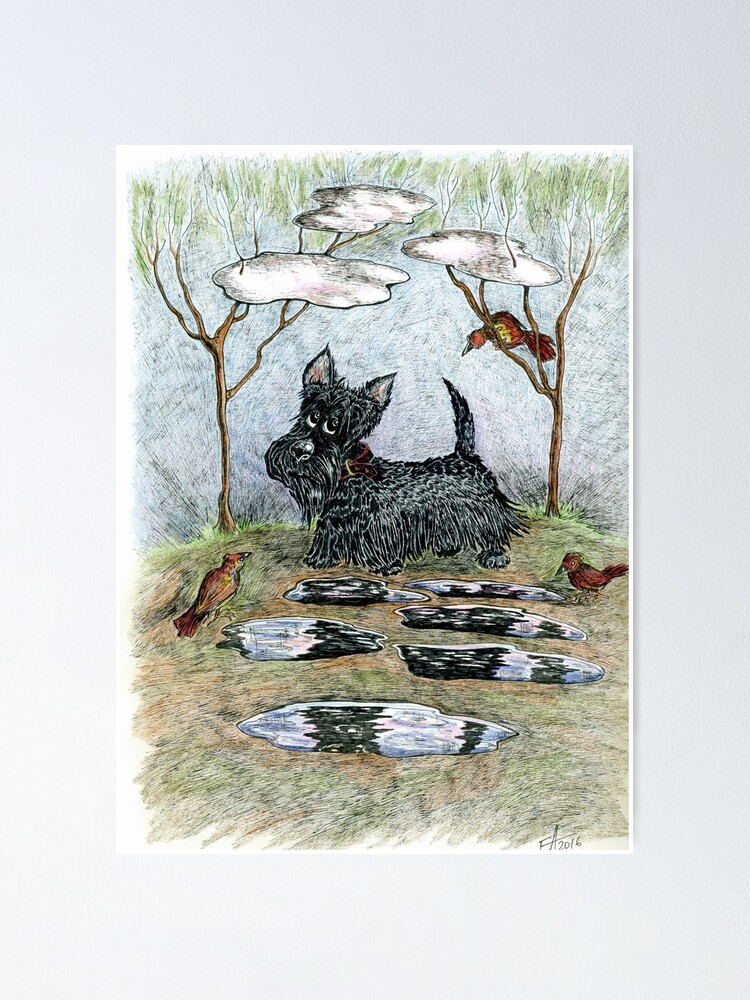The image is a detailed illustration on white paper set against a grayish-white background. The medium appears to be pencil, possibly supplemented with crayon, paint, or markers. At the heart of the scene is a Scottish terrier, characterized by long black hair, a distinct long beard, and pointy ears with a hint of pink, standing on a green hill. His tail is raised, and he gazes intently over the terrain. In the foreground, scattered around the hill, are patches of puddles mixed with black and gray rocks. To the right of the dog, a red bird drinks from one of these puddles, while a red and yellow bird to the left peers curiously at the Scottish terrier. The backdrop includes two brown trees sparsely adorned with green leaves, suggesting the season is changing. Above, a partly cloudy blue sky stretches out, contributing to the tranquil ambiance. The grassy hill itself is a mix of green and brown, varying in length. A discrete detail, a signature reading "FA 2016," is located at the bottom right corner of the artwork.